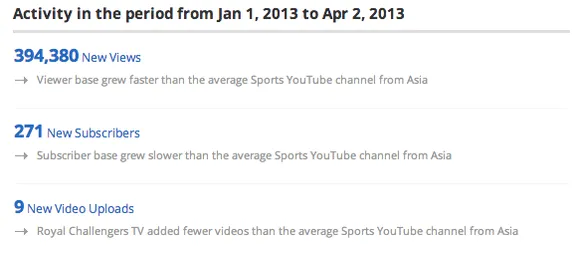**Detailed Performance Summary of Royal Challenger TV – Q1 2013**

This screenshot captures the performance metrics for Royal Challenger TV from January 1st, 2013 to April 2nd, 2013. During this period, the channel garnered 394,380 new views, which significantly outpaced the growth rate of the average sports YouTube channel from Asia. However, while the channel attracted 271 new subscribers, this growth was slower compared to the subscriber acquisition rate of these average Asian sports channels. Additionally, Royal Challenger TV uploaded a total of 9 new videos, a figure lower than the average number of video uploads by its Asian counterparts in the sports segment.

The screenshot features these key metrics in blue text set against a white background, with supporting information in gray type. The data highlights the channel's strengths in viewer engagement and identifies areas of potential improvement in subscriber and content growth.